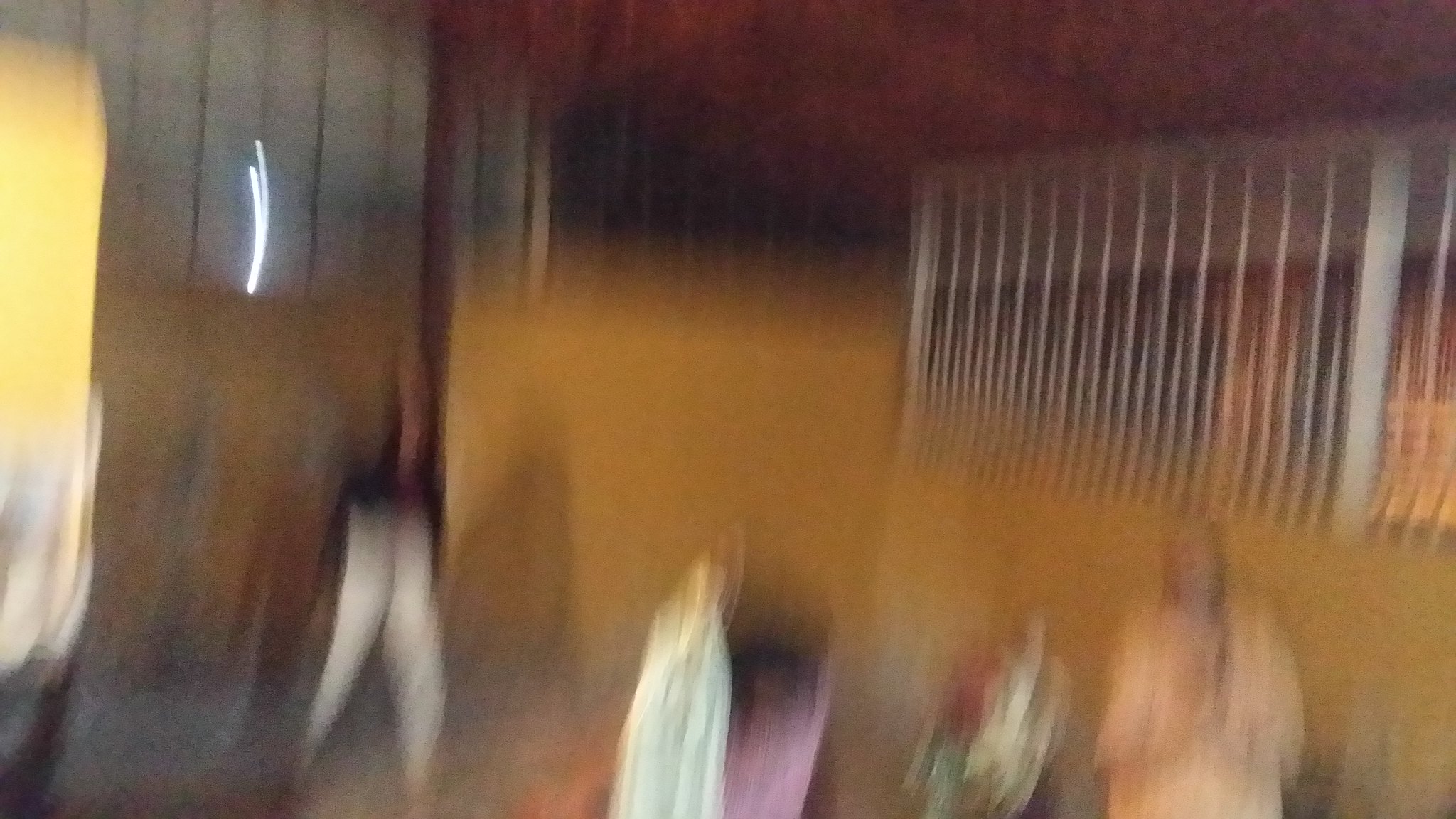The image, taken from a first-person perspective and likely in motion given its horizontal orientation and extreme blurriness, depicts an outdoor nighttime scene with notable architectural features. Dominating the scene are orange walls connected by white metal bars that match the height of the walls. To the left, a building with tall windows or a metallic reflective surface can be seen, extending into the background where another brownish structure with windows appears near a yellow-lit door. 

In the foreground, at least two indistinct figures are visible. On the lower right side, a woman appears to be wearing an oversized hoodie. Slightly behind and to her left is another woman with long black hair dressed in white pants that seem to distort her appearance due to the blurriness; she appears half-crouched as if in mid-motion. Additionally, several statues are discernible near the base of the orange wall: one character in a white gown, another with a mix of green, white, and red colors, and a third in a large orange robe. The scene is further enclosed by a high fence on the far right, stretching to the ceiling. The entire image suffers from severe graininess and distortion, making specific details challenging to pinpoint.